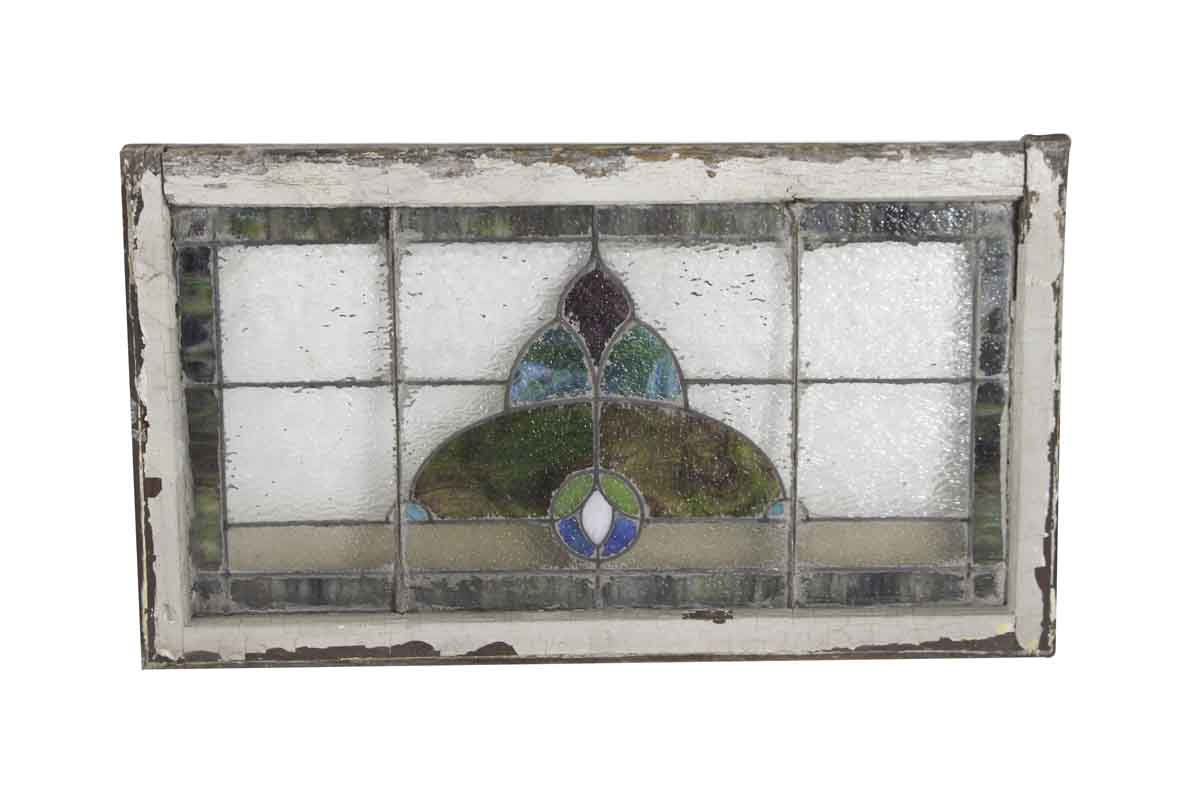The image depicts an extreme close-up of what appears to be a stained glass window set within a weathered wooden frame, originally painted white but chipped away to reveal the underlying brown wood. The main composition of the window features a slightly grayish-green border that encloses a grid of mostly white squares. At the center of the pane, there is a distinctive circular design at the bottom center which includes four vibrant leaf patterns: the top two leaves are green, the bottom two are blue, collectively creating a fifth white leaf pattern in the middle. Above this central circle, a dull green half-circle segues into two bluish-green petal shapes, and at the very top, a pointed dark petal shape, which is almost black, completes the design. The glass appears frosted and suggests a layered, multi-dimensional structure, with elements resembling mounds or cupolas, seamlessly blending into the overall motif of this historical artifact.